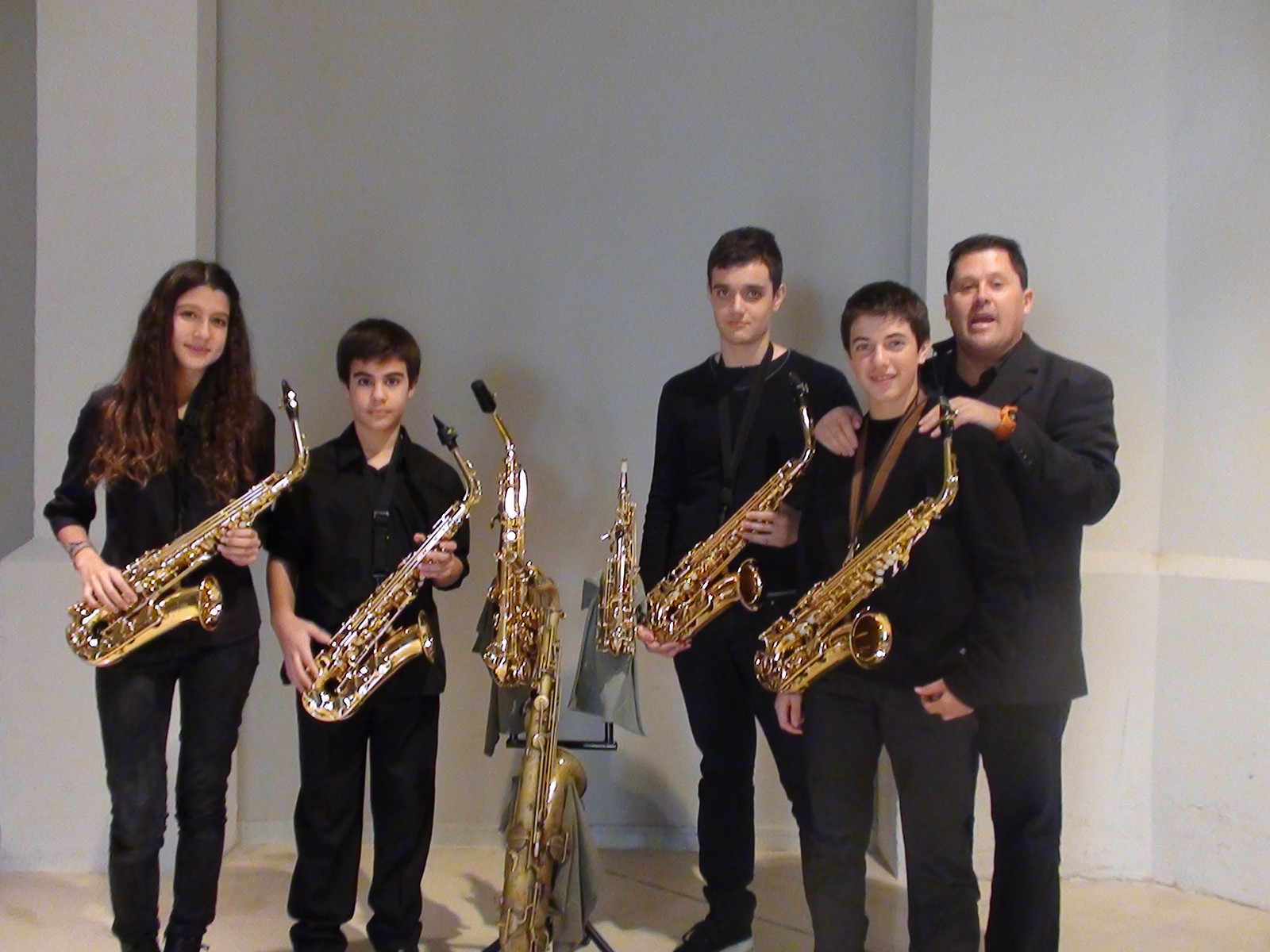In this photograph, five people are standing against a white wall with a grey door visible behind them. They appear to be part of a group, possibly a school band or a saxophone club. On the far left is a woman with long brown, curly hair reaching about six inches past her shoulders. She is dressed in all black and is holding a saxophone. Next to her stands a younger boy, also in black, who is about half a head shorter than her and is holding a saxophone as well. 

In the center of the image, there is a display case containing various brass instruments: a saxophone on the left, a trumpet in the middle, and a French horn on the right. To the right of this case is another young man in black, who is the tallest of the group, standing about a quarter of a head taller than the girl. He is also holding a saxophone. 

Next to him stands another young man, shorter than the tallest boy by about half a head, and he has a saxophone strapped around his neck. Behind this young boy is a middle-aged man, dressed similarly in all black with a gold watch peeking out from his suit, with his hands resting on the boy’s shoulders, suggesting a supportive or guiding role. The group is looking towards the camera, possibly in a posed formation for a photo-op illustrating their association with music.